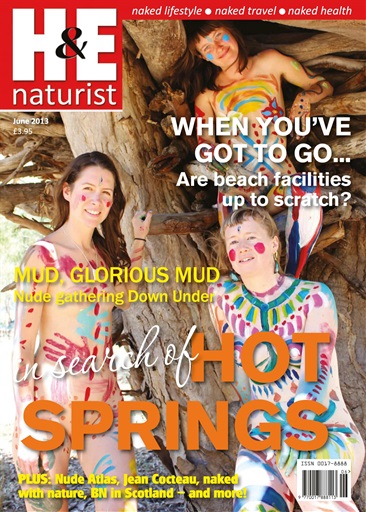The magazine cover of H&E Naturist features a vibrant and eye-catching image of three women posing in front of a large tree, their bodies adorned with colorful paint that artistically conceals their nudity. Across the top of the cover in a bold red background, white text reads, "Naked Lifestyle, Naked Travel, Naked Health." Additional prominent text throughout the cover highlights various articles, such as "When You've Got to Go, Our Beach Facility Is Up to Scratch" in white, "Mud, Glorious Mud, Nude Gathering Down Under" in yellow on the left, "In Search of Hot Springs" with "hot springs" in orange in the middle, and at the bottom, "Plus Nude Atlas, Jean Cocteau, Naked with Nature, BN in Scotland, and More." The vivid body paint includes striking designs like a rainbow painted across one woman’s chest and circles on their cheeks, adding to the artistic and naturist theme of the magazine. An ISBN label is visible at the bottom, underscoring its publication authenticity.